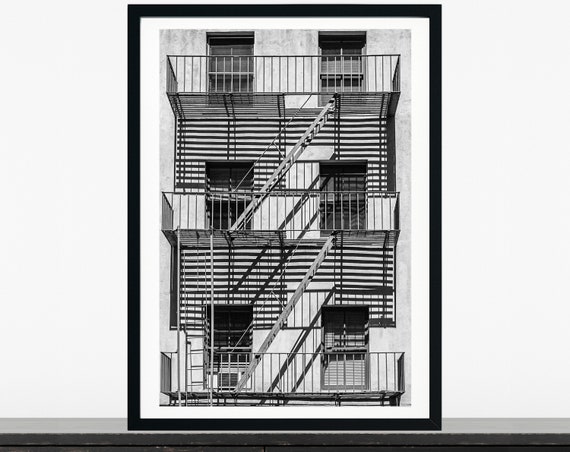The photograph, depicted in black and white, is framed in a sleek black frame with a white border and rests on a dark-colored platform. The captured image showcases a side view of a pristine white, three-story building, adorned with six evenly spaced windows - two per floor. Each window is protected by iron grating. The building features complex, geometric fire escapes, crafted from closely spaced metal bars which cast intricate shadows onto the building. These fire escapes consist of metal staircases and iron railings, leading down from the top floor to the second, and are interconnected by ladders on the outer left side of each railing, continuing down to the next level. The photograph's composition emphasizes the stark contrast and repeating patterns of the ironwork against the light building façade.